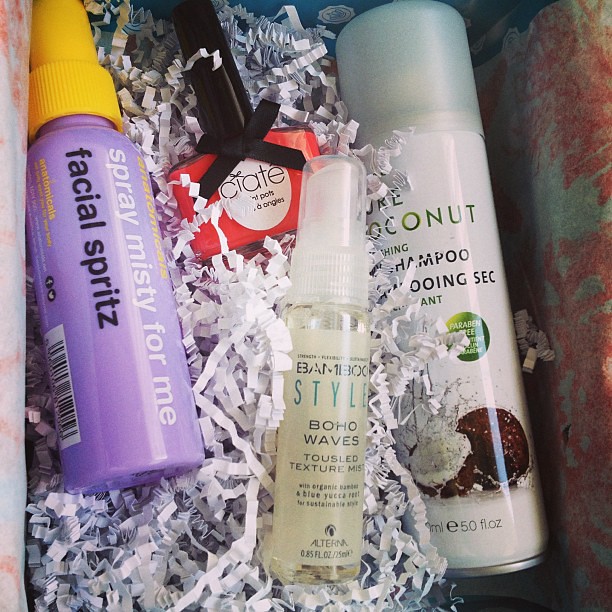This beautifully curated gift basket features a range of luxurious beauty and personal care products. At the forefront is a bamboo-styled Boho Wave Tassel Texture Mist, infused with organic bamboo and blue yucca for a sustainable, effortlessly chic hairstyle. A rejuvenating facial spritz promises to refresh and hydrate your skin throughout the day. Adding to the tropical charm, a coconut-scented shampoo transports your senses to an island paradise with each wash. The basket is adorned with vibrant confetti, lending a festive touch to the array. This exquisitely presented gift basket is brimming with pampering essentials designed to clean, nourish, and leave you smelling delightful.